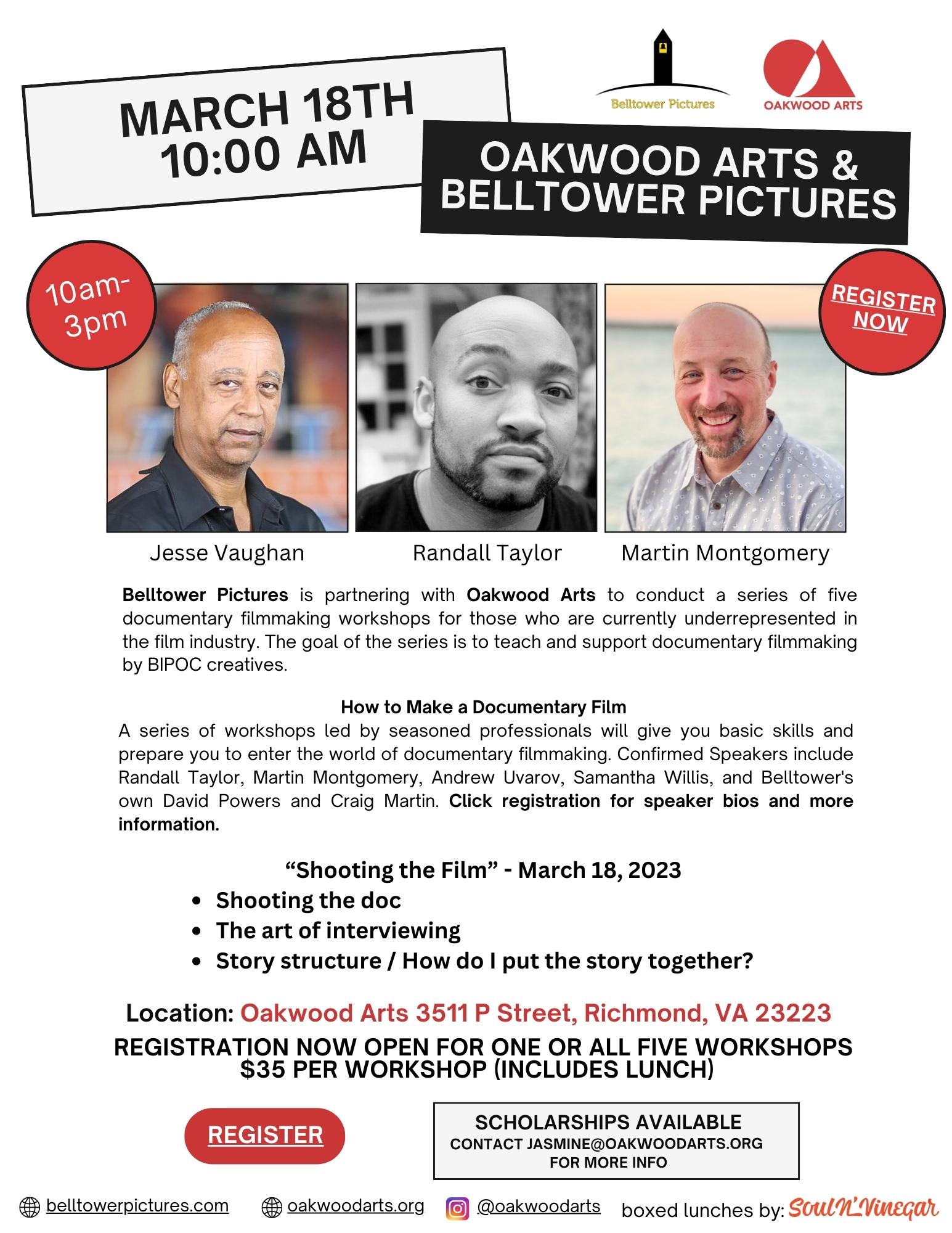This detailed flyer announces a documentary filmmaking workshop on March 18th, 2023, from 10 a.m. to 3 p.m., organized by Oakwood Arts and Belltower Pictures. At the top, the flyer prominently displays the event date, time, and the logos of both organizations. The event aims to teach and support documentary filmmaking, particularly for BIPOC creatives who are underrepresented in the film industry.

The workshop will cover various topics, including "Shooting the Film," "The Art of Interviewing," and "Story Structure: How to Put the Story Together." It's part of a series of five workshops designed to provide basic skills for entering the world of documentary filmmaking. Featured speakers include Jesse Vaughn, Randall Taylor, and Martin Montgomery, whose photos are displayed on the flyer. Vaughn and Taylor are identified as African American, while Montgomery is noted as white. 

The location for the event is Oakwood Arts, 3511 P Street, Richmond, Virginia, 23223. Registration for the workshops is now open, with a fee of $35 per workshop, which includes lunch provided by Sol & Vinegar. Additionally, scholarships are available for those in need, with more information accessible via a contact email. The flyer includes a call-to-action button to register and social media links for both organizing entities.